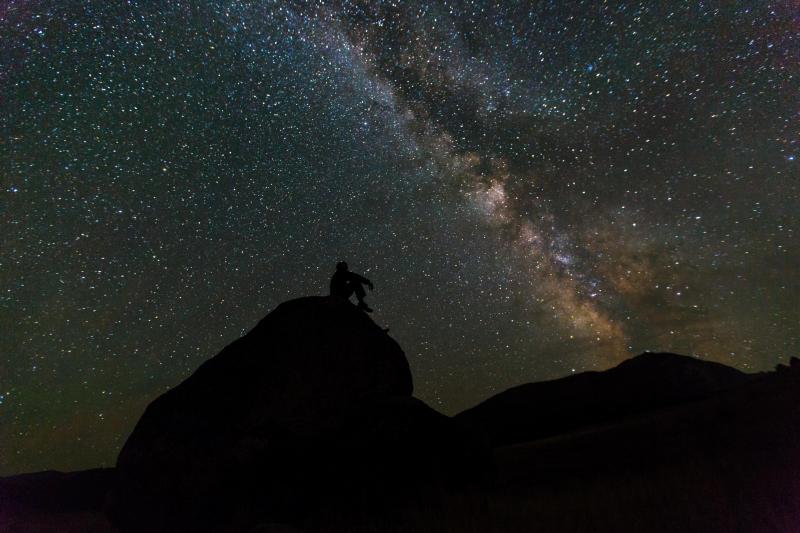This stunning nighttime image captures a silhouetted figure seated atop a large, shadowed rock formation on the left – the highest point in the foreground. The person, whose gender is indeterminate, sits with knees up and arms resting on them, gazing up at the awe-inspiring night sky. The backdrop is a mesmerizing tapestry of countless stars in various colors, evoking a northern lights-like ambiance with hues of blue and brown. Stretching diagonally from the horizon to the zenith is a light-colored streak, possibly a cloud or an atmospheric phenomenon, adding to the celestial splendor. Despite the rocks appearing as dark, indistinct shapes due to the absence of light, the overall scene is undeniably beautiful and serene.